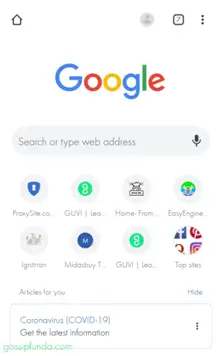The image depicts a mobile web browser interface dominated by a faint, diagonal watermark that reads "watermarked" with only partial visibility, showing portions of the letters "A", "T-E-R-M-A-R-K", and a fragment of "E". Positioned behind this watermark is the Google logo, highlighted in its characteristic colors: blue, red, yellow, and green.

The primary functionalities of the web browser are displayed prominently. Users are given the option to search for new web addresses via a microphone icon or a text box. Below the search bar, a history of recently visited sites is visible. These sites include ProxySite.com, Gov, Home, Local Engineer, Engstrom, Midsbury, GUVI, and Top Shelf, indicating a diverse range of previously accessed content.

Further down, there is a section titled "Articles for You," featuring a prominently displayed article about "Coronavirus (COVID-19)," encouraging the user to "Get the latest information." Adjacent to this section on the right, an ellipsis icon hints at additional settings or options available for user customization.

The background of the interface is primarily white or light, creating a clean and uncluttered look. In the top left corner, there is a home button, while the top right corner displays an icon indicating multiple open tabs, with the number seven signifying the total tabs opened.

Intriguingly, in the lower left corner of the screen, green lettering spells out another watermark, which says "GossipLunda.com". Additionally, in the upper right corner, there is another set of circles forming an ellipsis, providing further settings adjustments.

Overall, the image captures a detailed snapshot of a mobile web browser interface with multiple functional elements and informational cues.